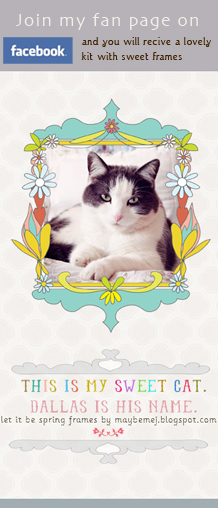The image features a promotional graphic for a Facebook page on a white background. At the top, a rectangular strip with a white font reads "Join my fan page on," followed by a blue square containing the text "Facebook" in white. To the right, in smaller black font, it states, "and you will receive a lovely kit with sweet frames." 

Below, the background transitions to a faint grey adorned with subtle white diamond shapes. The centerpiece of the image is a framed picture of a black and white cat. The cat has a predominantly black face with a white streak down the middle, white inside its ears, and a white chest, while the sides of its body remain black. The frame surrounding the cat is turquoise, embellished with white and yellow flowers. 

Underneath the picture, there is a decorative grey border with mirrored heart shapes. Between these borders, the text "This is my sweet cat" appears in rainbow colors, followed by "Dallas is his name" in pink. Finally, in black font, it reads, "Let it be spring frames by maybemej.blogspot.com".